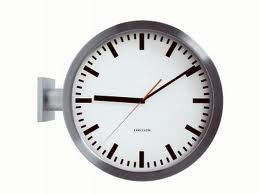The image features a wall-mounted clock that appears to be either double-sided or designed to be seen from different angles, with its mounting bracket clearly positioned on the left side. The clock face is oriented sideways, suggesting it attaches to a wall such that the 9 o'clock hour is where the mount is situated. The clock indicates a time of approximately 9:09, with the hour hand just past the 9, the minute hand just before the 10-minute mark, and the red, thin second hand around the 37-second mark. The clock's design includes no numerical indicators, only bold hour markers and dashed ticks at every 5-minute interval. The border and mount are a sleek gray or silver metal, and the clock hands are mostly black, except for the red second hand. Below the clock center, there's some small, unreadable branding. The face of the clock is white, contributing to the modern and minimalist aesthetic, possibly indicating that the image might be a computer-generated rendering or illustration rather than a photograph.